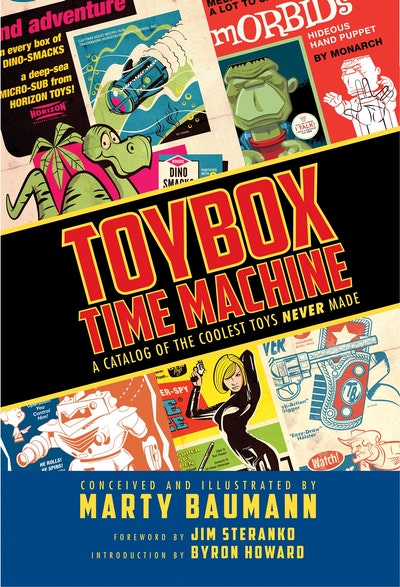The image showcases a vibrant, retro-style catalog cover titled "Toy Box Time Machine." Dominating the center is a black diagonal banner with bold red letters, outlined in yellow, proclaiming "Toy Box Time Machine." Beneath this title, in smaller yellow text, it reads "A catalog of the coolest toys never made." The top and bottom of the cover are framed with yellow strips, giving it a classic toy catalog aesthetic. 

In the upper left corner, obscured slightly by the edge of the image, you can glimpse the word "Adventure" in pink, situated above various intriguing toy illustrations. These include a green dinosaur beside a palm tree, a descending rocket emitting smoke, and a deep-sea microsub from Horizon Toys. 

The upper right corner features an orange background with the word "Morbids" in white. This section displays two images of a monstrous green hand puppet, one fully colored and the other a white outline with an extended hand. 

Near the bottom, nestled under the black banner, is an illustration of a vintage robot. Additionally, in one part of the middle section, there's a striking female character donned in a sleek black suit, blonde hair flowing, and holding a pistol aloft. Adjacent to her, a pistol in front of a holster is depicted, and in the lower corner, a red-inked outline of a cowboy leaning forward and gazing leftwards can be seen, accompanied by a red circle labeled "Watch."

At the very bottom, a blue banner with yellow letters credits the creators: "Conceived and Illustrated by Marty Baumann, Foreword by Jim Steranko, and Introduced by Byron Howard." The overall design exudes a nostalgic charm with its faded yet colorful palette, reminiscent of classic comic books and vintage toy advertisements, embodying the theme of fantastical, never-produced toys.